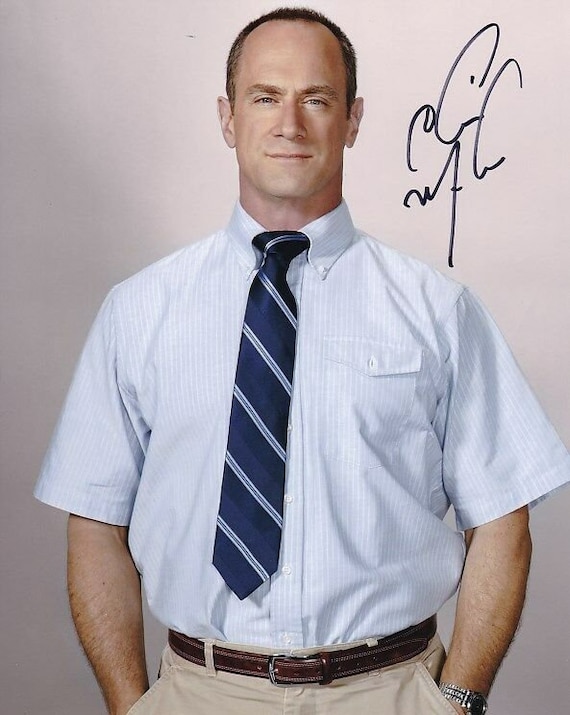This signed photograph features a male actor known for his roles in television series such as "Law and Order: Special Victims Unit" and possibly "NCIS" or an FBI-related show. He is a white male with very short brown hair and a high receding hairline. His expression is somewhat fierce and proud, yet he also has a slight smile.

He is dressed in a short-sleeved, light-colored dress shirt—reportedly white or light blue—with button collars, paired with a blue and silver striped tie characterized by slanted white and blue lines. He is also wearing khaki pants secured by a dark brown leather belt and a metallic silver watch. His hands rest casually in his pockets.

The photograph has a peculiar signature in the upper-right corner that may need a handwriting analyst to decipher. The actor stands against a neutral gray background with some top lighting, suggesting this might be a promotional image, perhaps distributed to fan clubs or taken on a film set.